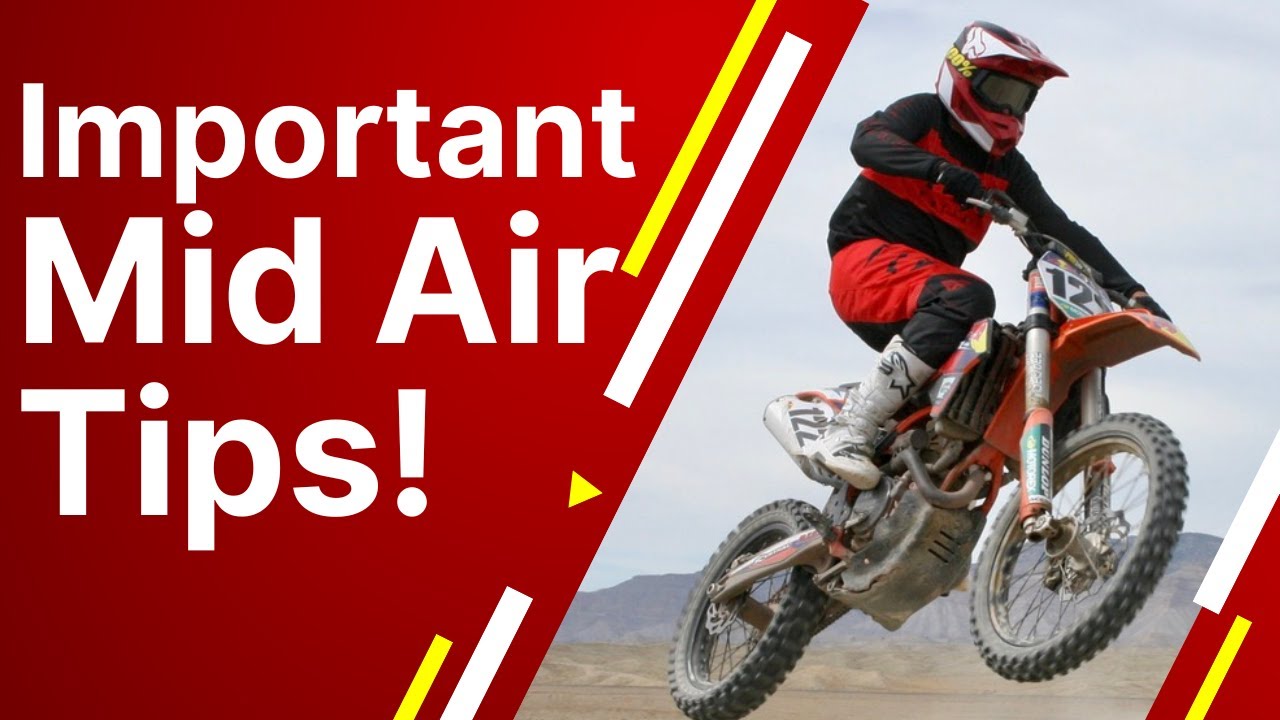The image is a detailed poster or title page, prominently divided by a sharp diagonal line from the right to the left. On the left-hand side of the line, the background is a solid red color with the text "Important Mid-Air Tips!" written in white, chunky font, with each word's initial letter capitalized and an exclamation point at the end. Adjacent to this, there are parallel white lines resembling road lines, with a yellow-greenish triangle nestled between two of the lines and two yellow stripes on top, potentially indicative of a digital button.

On the right side, there is a dynamic image of a motocross rider in mid-jump, emphasizing the "mid-air" concept from the text. The rider, wearing a red and black suit with white, silver, and black protective gear, and a helmet with a shaded visor, is depicted in action. The motorcycle itself has a red fender and bears a competition number that starts with 120, although the last digit is partially obscured and could be a 2, 4, or 9. The background also features mountains, accentuating the scene's adventurous and competitive nature.